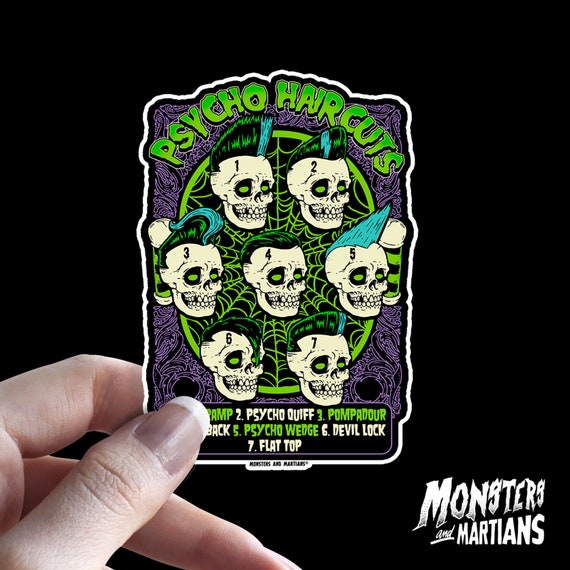A woman's hand, with a French tip manicure, holds a sticker or trading card with jagged edges. The card features a vibrant color scheme of purple, green, black, white, and light blue. At the top, in green text, it reads "Psycho Haircuts." The main design consists of seven white skulls, each with blue hair styled in various punk rock-inspired haircuts. These styles, numbered on the skulls’ foreheads, are Psycho Quiff, Pompadour, Devil Lock, Flat Top, and Psycho Wedge. The fingertip partially obscures the names of haircuts one and four. Below the skulls, in white text on a black background, the names of the haircuts are listed. The card is inscribed with "Monsters and Martians" in the lower right-hand corner.